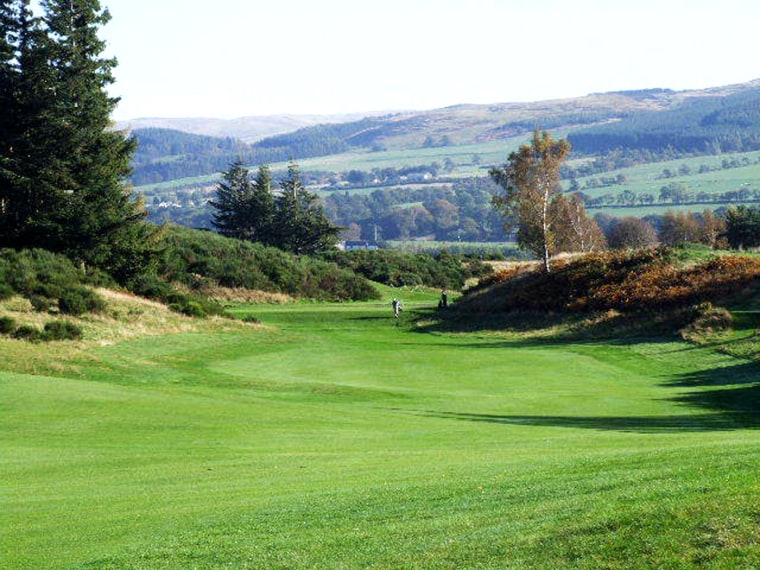The photograph captures an expansive outdoor scene that is likely a golf course, evident from the meticulously manicured, vibrant green grass stretching broadly across the foreground. This central green plain resembles a fairway, bordered on both sides by gentle hills. The hill on the left is adorned with lush green bushes and topped with evergreen trees, creating a verdant landscape. In contrast, the hill on the right features short, brownish vegetation, interspersed with small deciduous saplings, likely birch trees with foliage turning brown, indicative of the fall season. The distant horizon reveals alternating rows of rolling hills and grassy patches, culminating in a line of low, flat mountains beneath a pale blue sky. In the hazy distance, a golfer dressed in blue, possibly with another figure in shadows nearby, can be seen walking down the fairway, adding a subtle presence of human activity to this serene and pastoral setting.